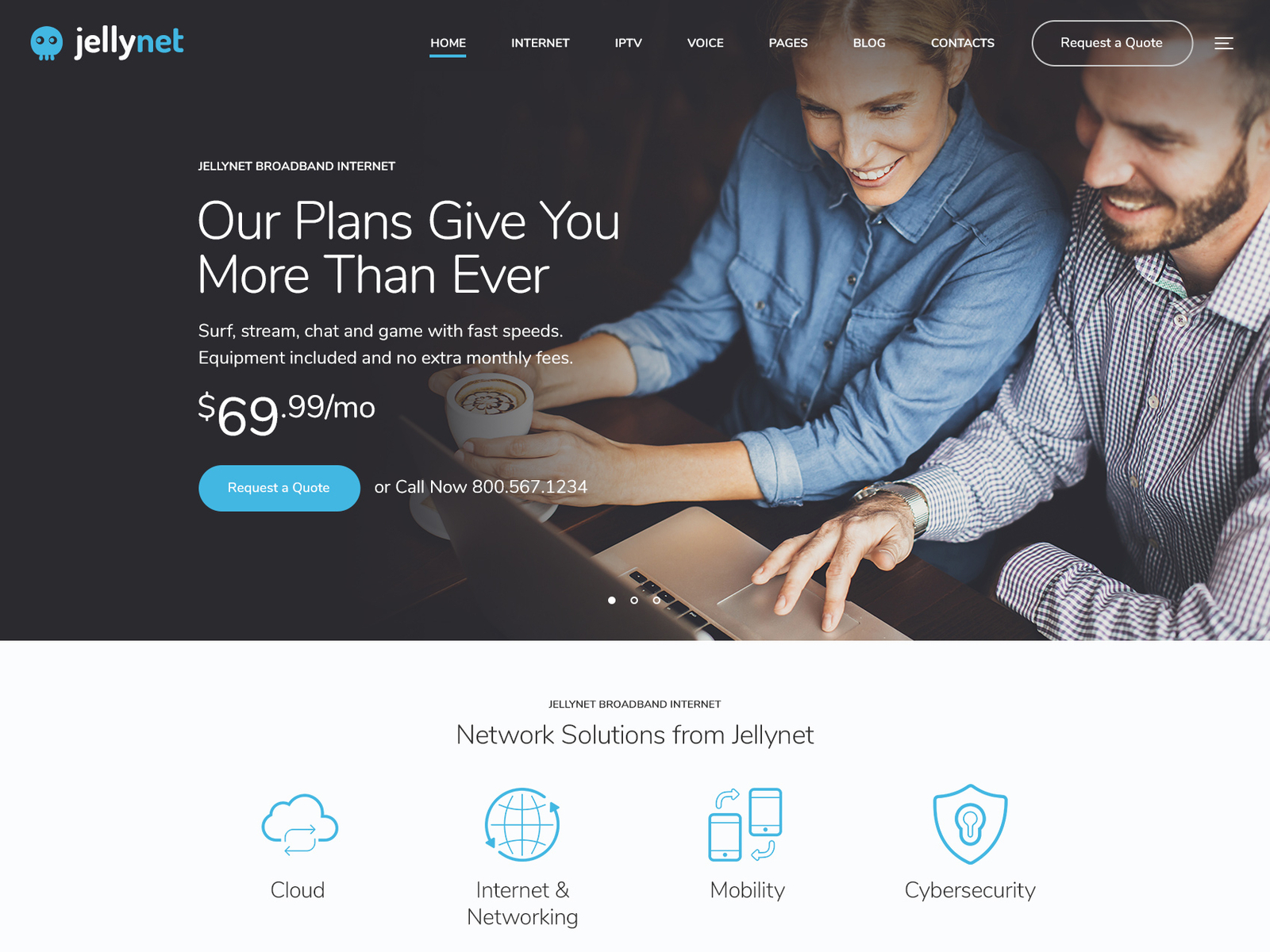The top section of the image features an advertisement banner prominently displaying the JellyNet logo in white and light blue. Below the logo is a navigation taskbar with clickable links labeled: Home, Internet, IPTV, Voice, Pages, Blog, and Contacts. Adjacent to these links is a blue button reading "Request a Quote."

Beneath the navigation bar is the main promotional text which highlights the comprehensive services provided by JellyNet: "JellyNet offers Broadband Internet and IPTV more than ever before. Enjoy surfing, streaming, chatting, and gaming at fast speeds. All equipment is included with no additional monthly fees for just $69.99 a month." Another blue "Request a Quote" button appears here alongside a contact number for immediate assistance, "Call Now at 800-567-1234."

The central visual element of the image shows a young, smiling man and woman. The woman holds a cup of coffee while the man is engaged with a laptop, both appearing content and connected. The ambiance suggests a professional yet relaxed environment enhanced by JellyNet’s reliable service.

The bottom section reiterates JellyNet's commitment to comprehensive broadband solutions, listing their expertise in Network Solutions, Cloud Services, Internet Networking, Mobility, and Cybersecurity: "JellyNet: Broadband Internet, Network Solutions from JellyNet, Cloud, Internet Networking, Mobility, Cybersecurity."